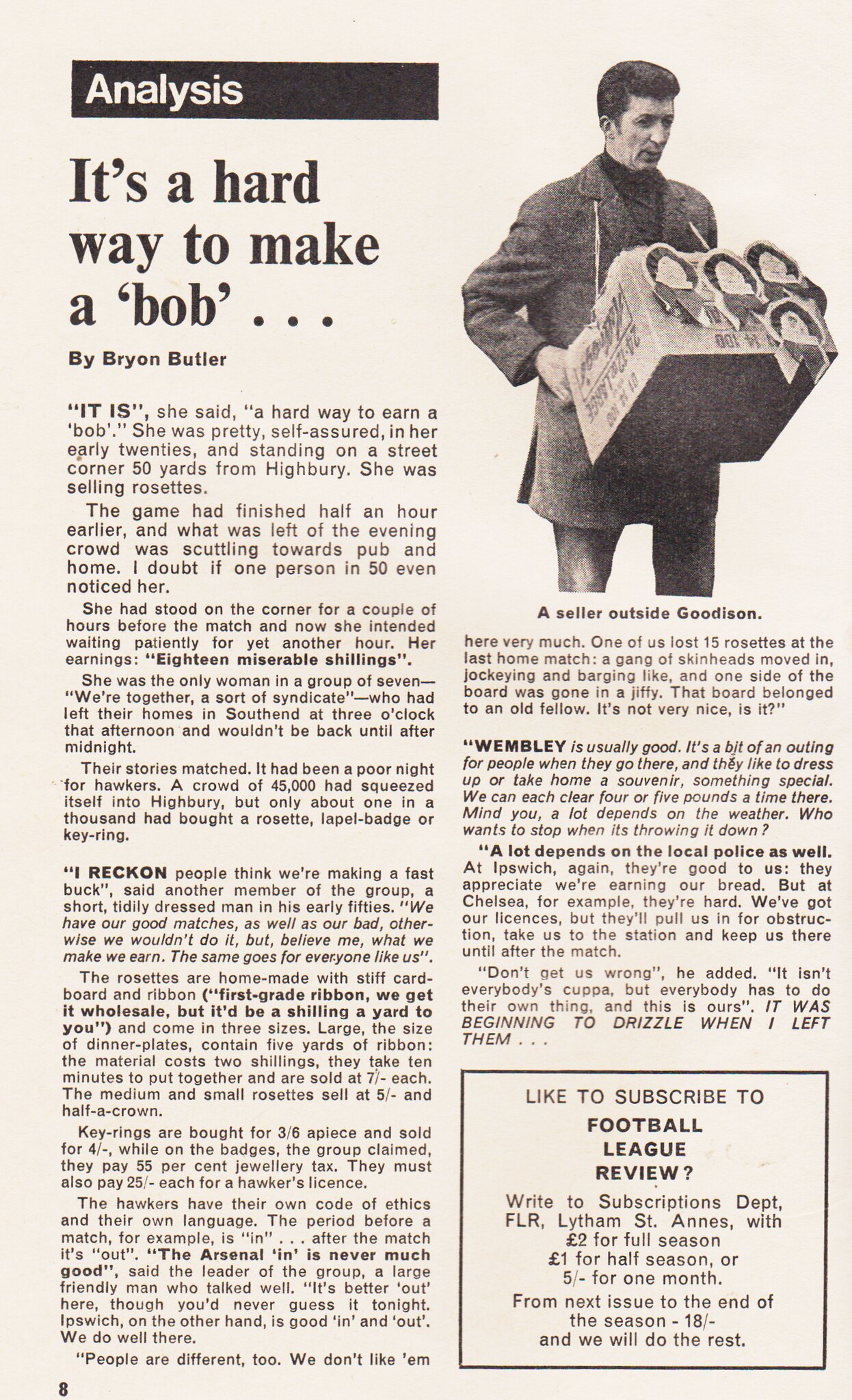This black-and-white page from a game day magazine or program, divided into two columns, features a detailed article by Brian Butler titled "It's a Hard Way to Make a Bob." At the top left of the left column, a black bar bears the white text "Analysis." Below it, the article begins with an anecdote about a confident young woman selling rosettes near Highbury. Accompanying the article is a black-and-white photo of a man with black hair, dressed in a coat and jeans, carrying a box with indistinguishable items. The caption reads, "A Seller Outside Goodison." The article, spanning thirteen paragraphs, provides an in-depth analysis of the difficulties in earning a living through street vending. At the bottom of the right column, a subscription box offers readers the option to subscribe to the "Football League Review" for $2 per full season or $1 per half season.